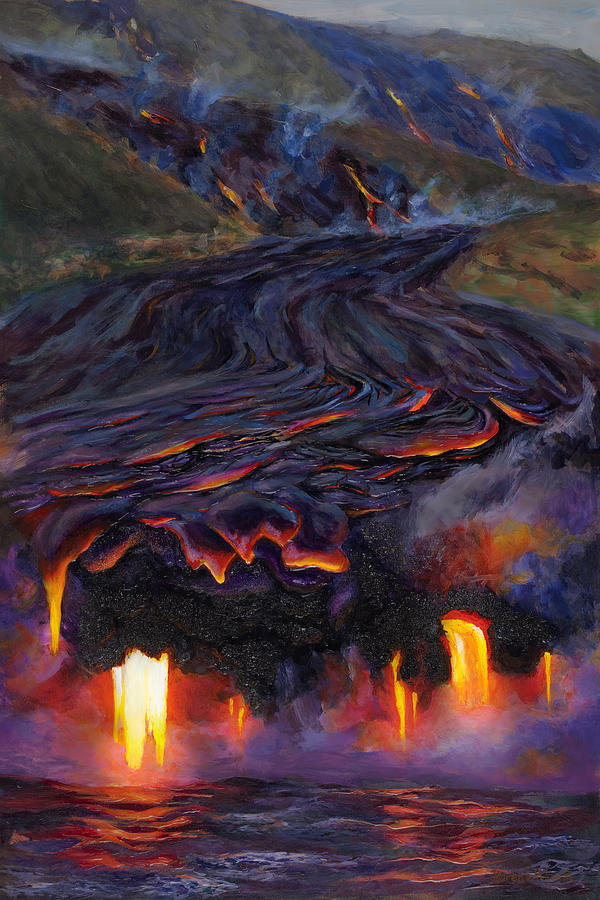This detailed painting vividly captures the dramatic scene of a fresh lava eruption cascading down a multi-tiered hill or small mountain. The composition is divided into three distinct sections, starting from the top right where the molten lava begins its descent. The vibrant bright oranges and yellows of the lava contrast starkly with the jet black areas where it has cooled, creating a striking visual effect. As the lava flows down the hill, it reaches the center of the painting and eventually meets the sea at the bottom. Here, the extreme temperature difference between the lava and the water generates a plume of white mist and spray, artistically rendering the intense heat exchange. The painting's upper regions display scattered, coal-like black tops caused by the air cooling the lava, interspersed with veins of glowing orange and yellow that hint at the ongoing volcanic activity beneath. This masterful use of color and texture not only portrays the raw power of nature but also brings to life the awe-inspiring moment of lava meeting the ocean.